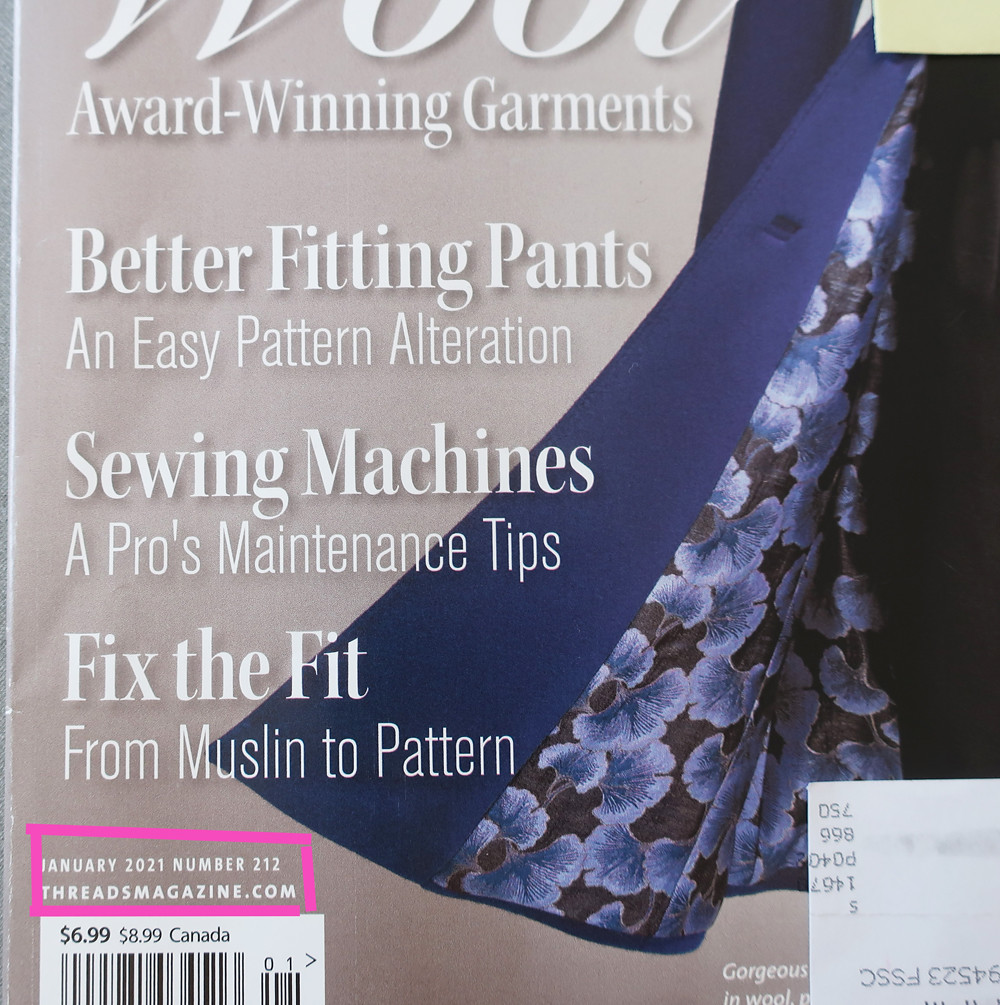The image depicts the front cover of Fred's Magazine, specifically the lower left quadrant. It features a stunning blue, ankle-length coat with a black and blue flower pattern lining inside. White text in a blue box reads, "January 2021, Number 212, Fred's Magazine." Additionally, there is a pink background with white text detailing award-winning garments, better fitting pants, easy pattern alterations, and sewing machine maintenance tips. A receipt is visible on the lower right, and the pricing information states $6.99, or $8.99 in Canada. The image composition suggests the objects are hanging flowy from the top right corner, emphasizing the fashion-forward aesthetic of the magazine's cover.